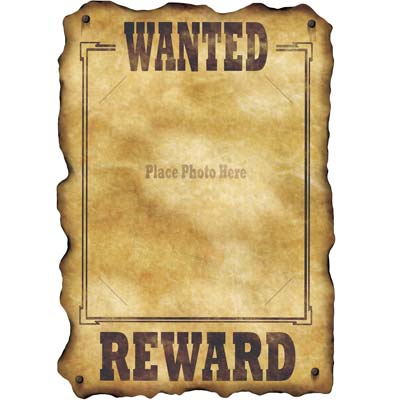This is an image of a Wanted poster that appears to be a piece of computerized artwork. The poster has the appearance of an old, burnt piece of paper with irregular, charred edges that give it an aged look. Each of the four corners of the poster is secured by dark brown metal nails. At the top of the poster, the word "WANTED" is prominently displayed in capital letters in brown. Similarly, at the bottom, the word "REWARD" is also in capital brown letters, matching the size and style of the text at the top.

In the center of the poster, there is a rectangular frame bordered by black lines, intended as a placeholder for a photograph. Inside this frame, the text "PLACE PHOTO HERE" is written in smaller letters, suggesting that the poster template is unfinished and meant for customization. The meticulous details, such as the burnt edges, brown coloring of the letters, and the metal nails, all enhance its vintage and weathered appearance, although its pristine and unmarked condition indicates it is a digital creation rather than an actual aged document.